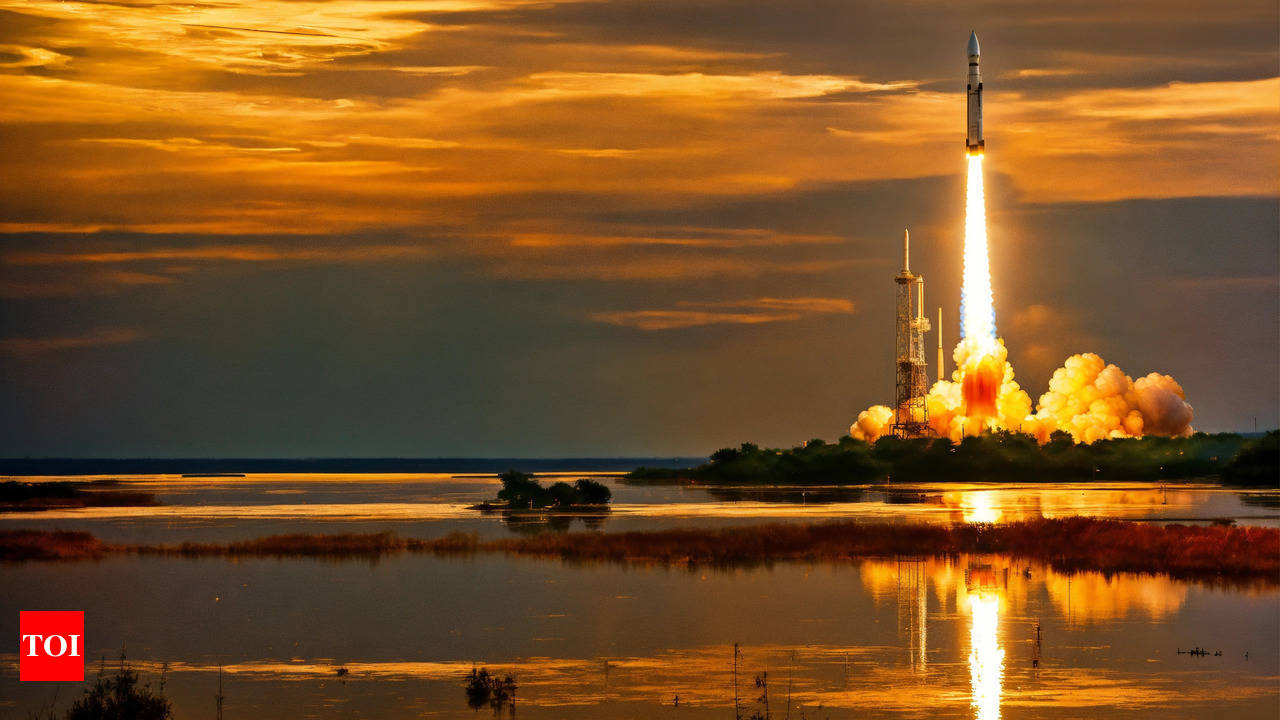The photograph captures a vivid scene of a dramatic rocket launch at dusk. In the bottom left corner, there's a red square with the letters "T.O.I." prominently displayed. The rocket, positioned slightly to the right, is blasting off with a trail of intense yellow fire and thick clouds of smoke billowing beneath it. The sky dominates the image, painted with stunning orange and gray hues as the sun sets, adding to the atmospheric tension. Below the rocket, a sprawling lake or body of water extends across the scene, reflecting the fiery launch, smoke, and surrounding marsh-like grasses. A towering structure stands next to the rocket, further emphasizing the scale and grandeur of the moment. The combination of natural beauty and human engineering prowess is breathtakingly captured, as the rocket ascends toward the sky, leaving behind a mesmerizing aftermath in the water's reflective surface.